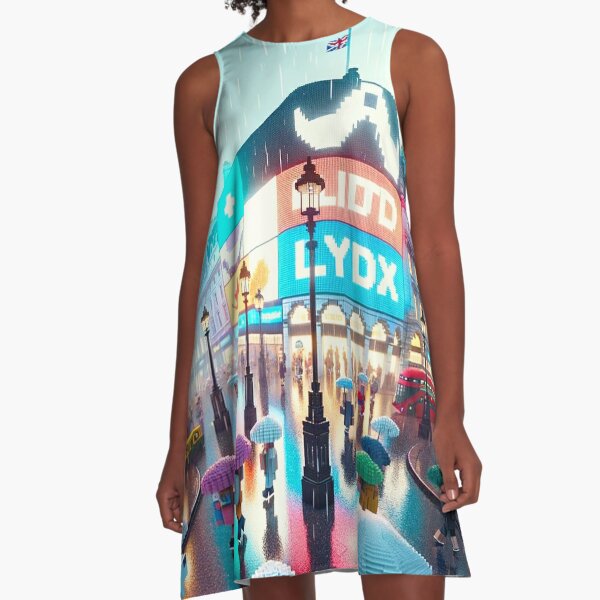This photograph features a woman with a dark brown complexion modeling a sleeveless shift-style sundress against a white background. The dress has a light blue base and vividly depicts a rainy city street scene that covers the entire fabric. Starting from the neckline, a British flag appears on the top right, alongside a detailed cityscape that includes a double-decker bus, various people with umbrellas, and multiple streetlamps. The umbrellas are checkered or solid in shades of blue, purple, green, and red. Among the five black wrought iron lampposts, one stands out by emanating a yellow light. The street scene indicates wet conditions with reflections on the ground, adding to the impression of rainfall. At the chest level, partially obscured by a lamppost, are banners displaying the letters "LYDX" and "LIDD" in a somewhat fragmented manner. The building in the backdrop has arched windows and a flag waving at its peak. The woman’s hair is visible at the top of the picture, although her face and anything below her knees are not shown. The dress accentuates a vibrant blend of faint pastel hues, making for a compelling and artistic representation of a bustling, rainy day in an urban setting.